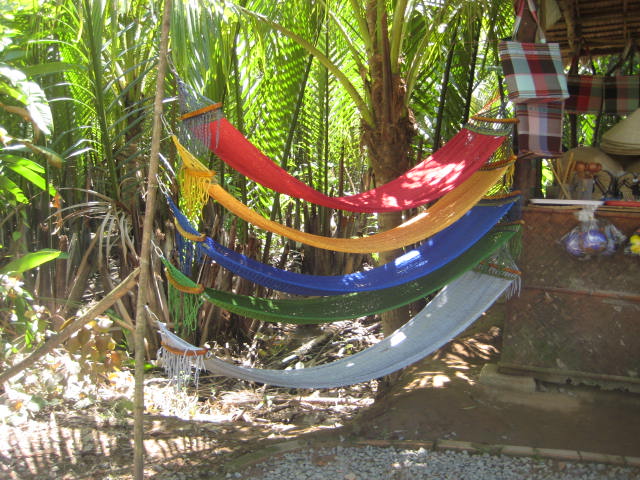This color photograph, taken during the daytime in a tropical outdoor setting, showcases a quaint cabana made of wooden sticks on the right side of the image. Inside the cabana, purses hang neatly. Stretching to the left is a single tree, its branches serving as one anchor point for an array of colorful hammocks, with the other end of the hammocks attached to the cabana. The hammocks are arranged in a vertical sequence with visible gaps between them: a red hammock at the top, followed by yellow, blue, green, and finally, a grayish-silver (or white) hammock at the bottom. The ground is covered in gravel and surrounded by tropical plants and tall palm trees. Shadows cast from the hammocks add depth to the scene, highlighting the serene and inviting atmosphere of this tropical haven.